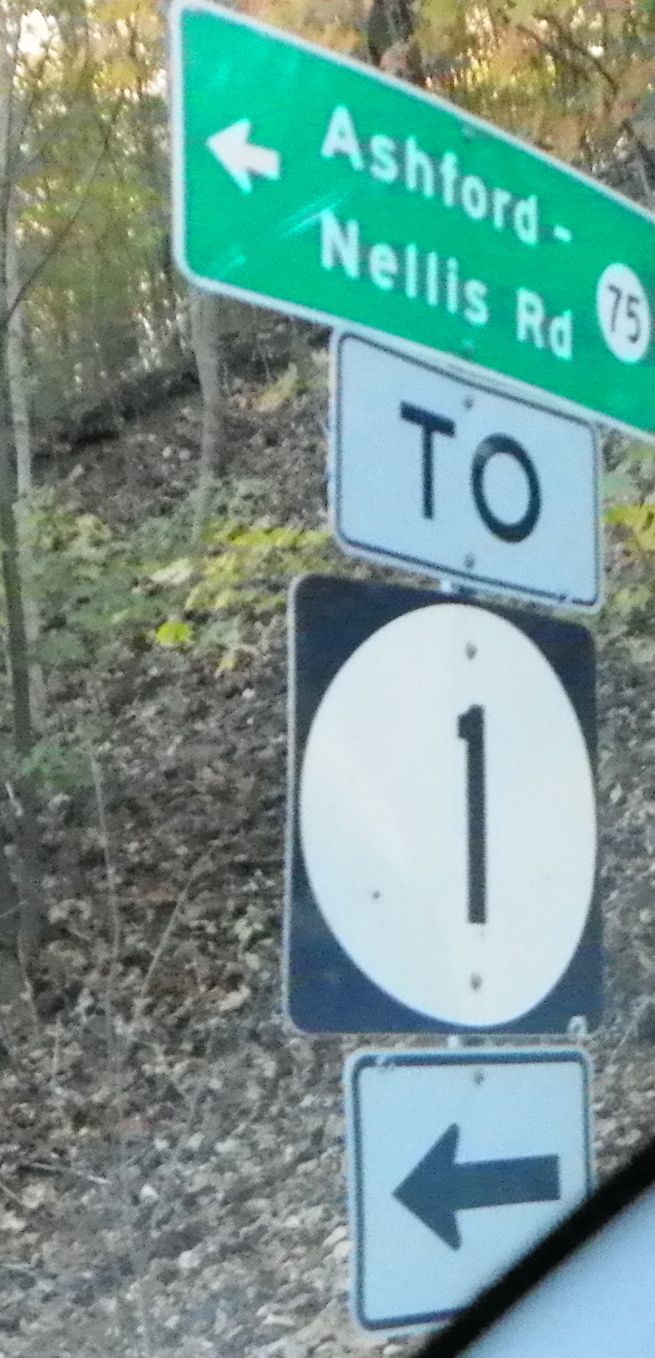This photograph captures a collection of road signs positioned on the side of a road, likely taken from inside a car judging by the diagonal slice of the car window at the bottom, represented by a small white triangle and a black line. The bottommost sign features a black arrow on a white background, directing traffic to the left. Just above it hangs a black square sign with a white circle, within which the number "1" is prominently displayed in black.

The next sign in the stack is a small white rectangle with a black border, bearing the text "2TO" in black letters. At the top of the array is a larger green rectangular sign with white text, showing the road name "Ashford-Nellis Road." This sign is adorned with a white circle on the right side containing the number "75" in black, and on the left side, a white arrow pointing to the left.

Surrounding the signs is a natural backdrop: a hill carpeted with layers of dead, gray leaves, typical of a late autumn or early winter scene. The upper section of the hill and portions throughout the middle exhibit clusters of greenery, including green and yellow-green leaves. The top of the hill is crowned with several trees, adding depth and context to the setting.